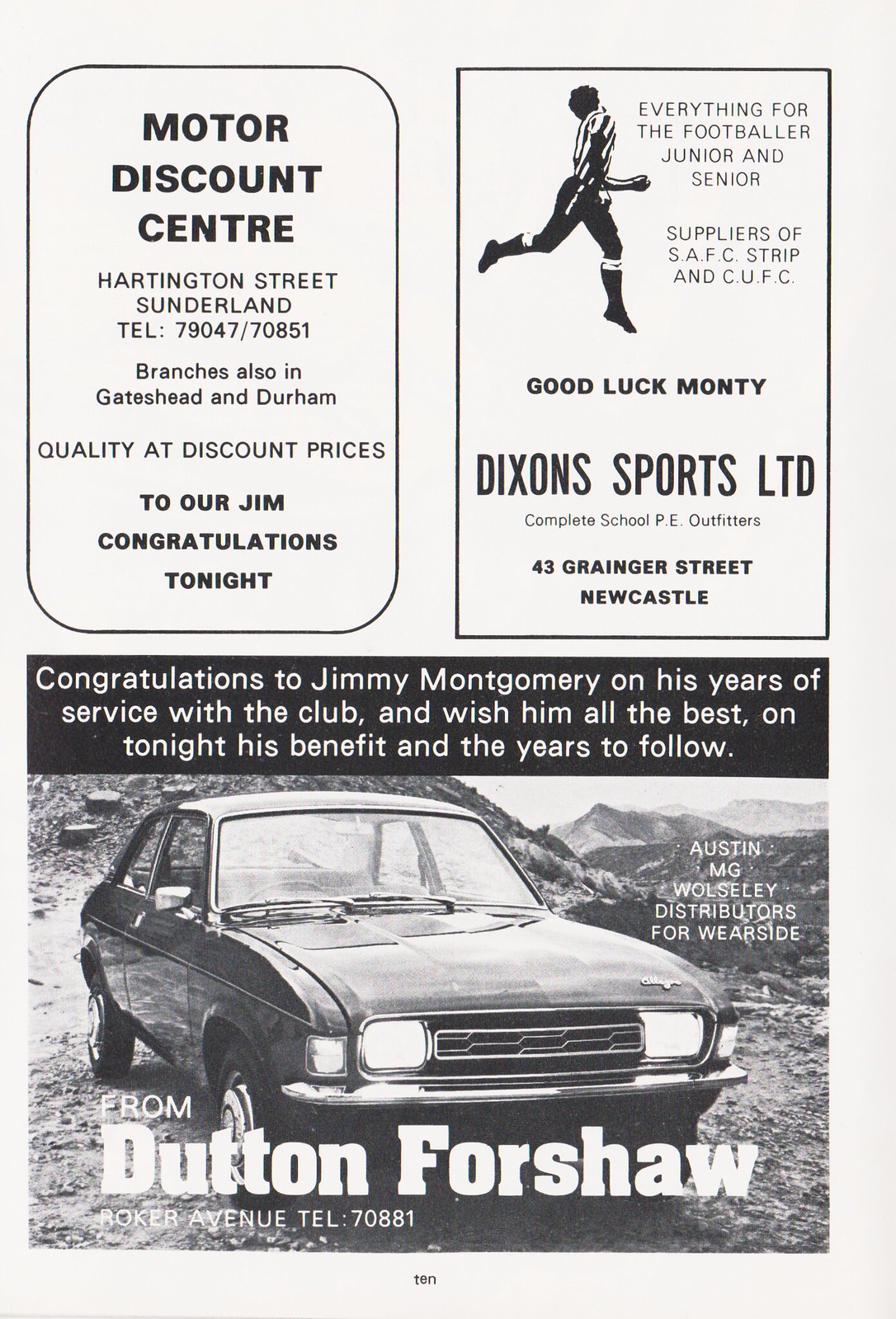The black and white image is a page from an old European football program, specifically page 10. The top half of the page features two advertisements. On the top left, an ad for Motor Discount Center provides a detailed address on Hardington Street, Sunderland, with additional branches in Gateshead and Durham. It reads, "Quality at discount prices," and includes a congratulatory message: "To our Jim, congratulations tonight." On the top right, Dixon Sports LTD advertises itself as a supplier for both junior and senior footballers, specifically mentioning SAFC and CUFC strips. The ad also wishes "good luck, Monty," and lists its location on 43 Granger Street, Newcastle. The bottom half of the page displays a car advertisement from Dutton Foreshaw located on Roker Avenue. It features a congratulatory message to Jimmy Montgomery, acknowledging his many years of service to the football club and extending best wishes for his benefit tonight and the future.